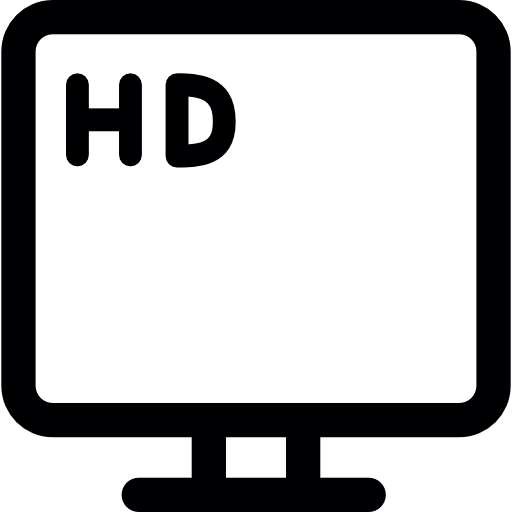The image depicts a stylized representation of an HD monitor on a white background. The monitor is a perfect square with rounded edges, bordered by a thick, black outline. Centrally positioned at the bottom, a short, rectangular stand with two vertical supports attaches to the monitor, creating a balanced and symmetrical look. The face of the monitor is white, featuring the bold, black letters "HD" prominently displayed in the upper left-hand corner. The entire illustration is rendered in black and white, giving it a clean and minimalist appearance. This image could serve as a stock photo for websites, a graphic on product packaging, or various other design purposes.